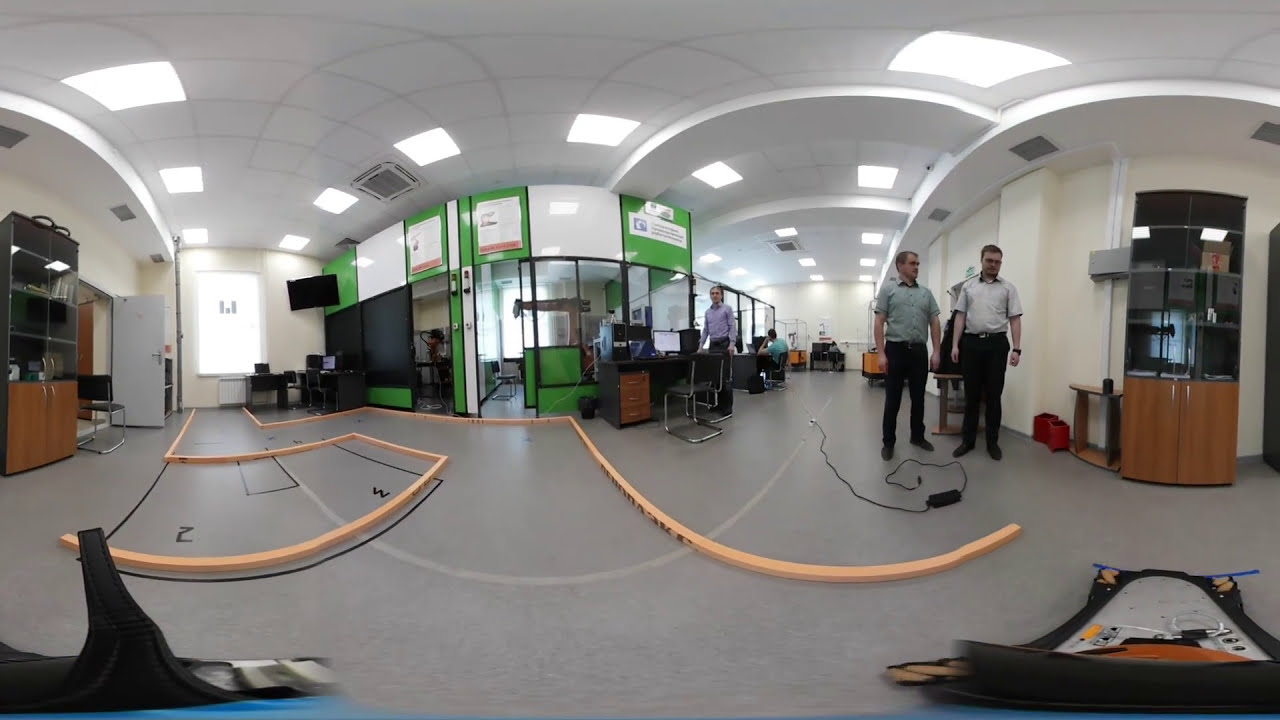This panoramic photograph captures the interior of what appears to be an office space, potentially under construction. The unusual camera lens creates intriguing distortions, making it seem as though the front door juts into the building. The setting is illuminated by fluorescent lights with covers, suspended from the white ceiling. The floor features a gray color, complemented by a curiously laid yellow path resembling dominoes, which seems to guide the placement of orange curved wooden beams that form a winding walkway.

Central to the image are green and blue walled offices with transparent glass windows, providing visibility into the interiors. There's a display of various objects: wood poles, desks, chairs, and display cases. Toward the left, a cabinet with a TV in one corner is visible, while more storage units and office furniture occupy other areas. Notably, the bottom half of the image appears more open, with scattered wood beams creating a somewhat natural placement.

Three men are present in the scene; two stand on the right side near a desk, dressed in business casual attire featuring black pants, and light-colored shirts in shades like lavender, light green, and white. A third person is seated further back. The entire composition, layered with its dynamic elements and static figures, suggests a transitional phase in the office's setup.